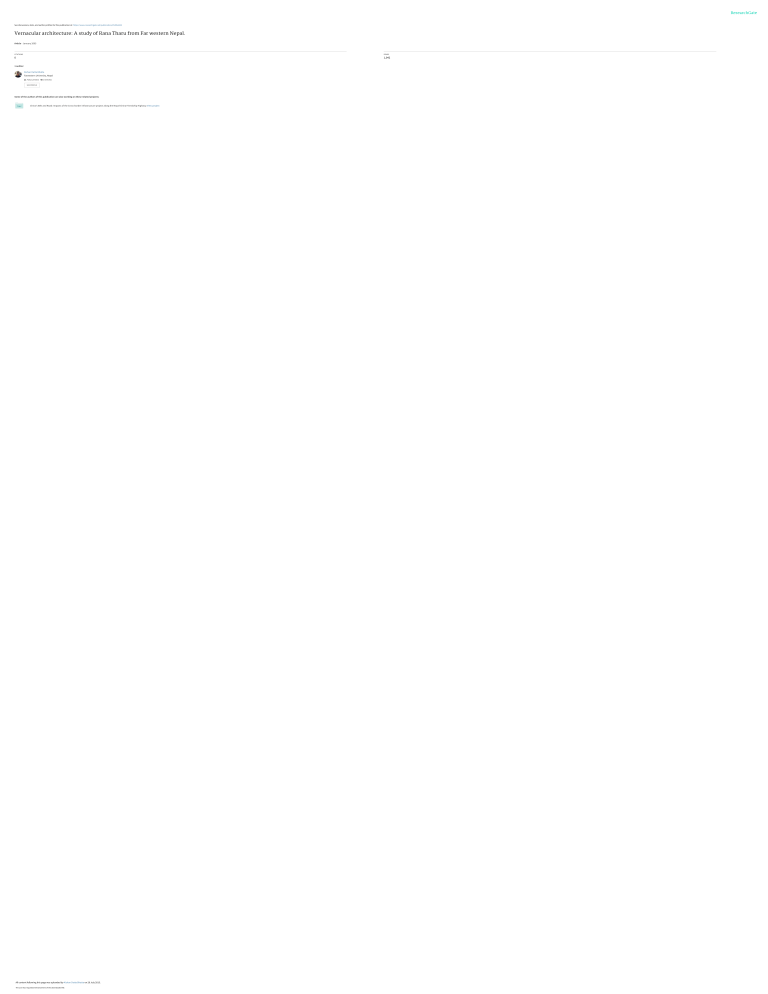The top-right corner of the image features a research key. The primary colors used in the text within the image are black and blue. The subject focuses on vernacular architecture, with studies conducted from the right, left, and center perspectives. A distinct line separates sections of the image, leading to additional text and blue elements throughout. The image also contains several paintings, characterized by white backgrounds, all interspersed with a mix of black and blue text, creating a visually engaging and detailed collage of architectural studies and artistic elements.